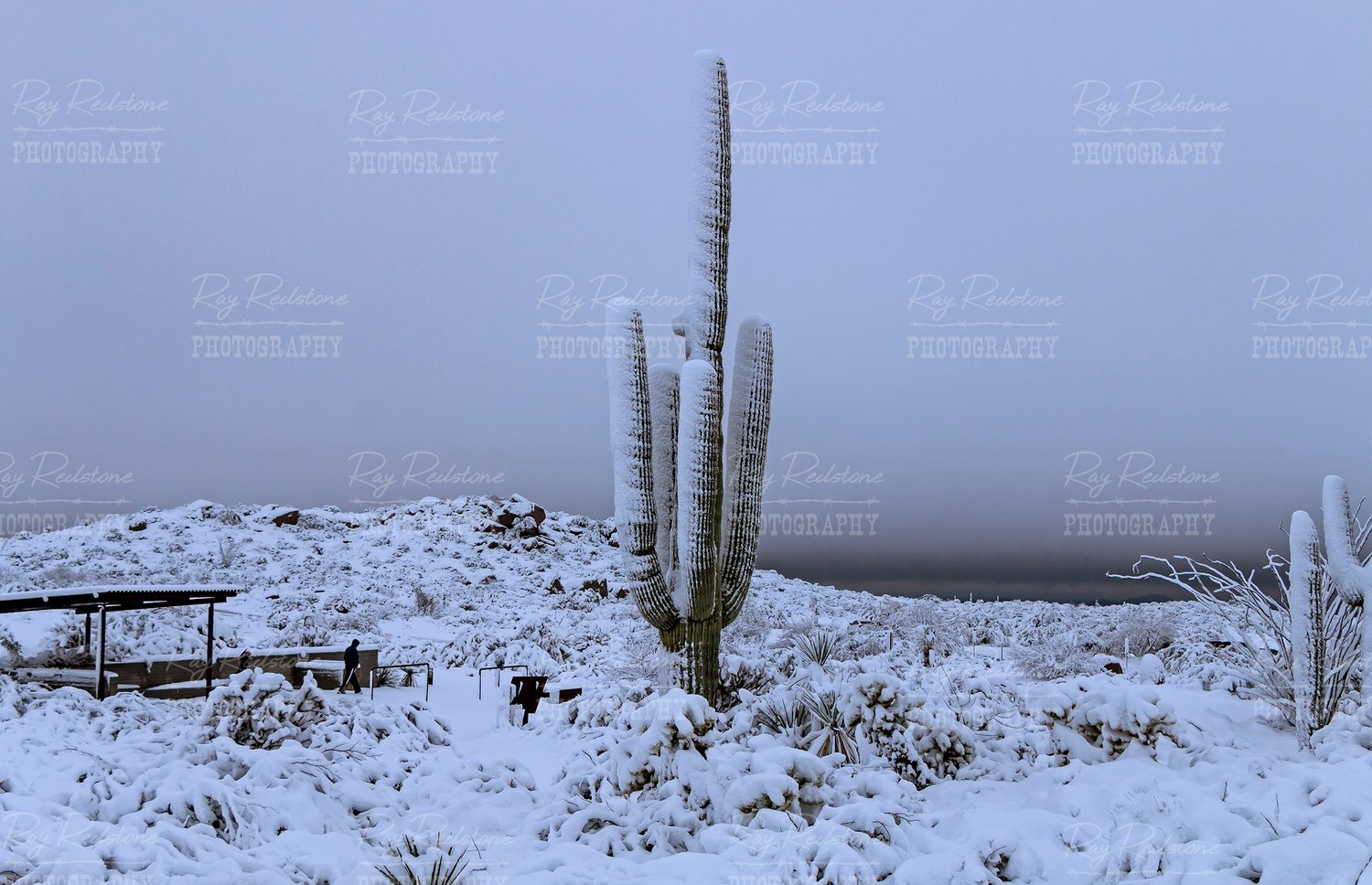This monochromatic photograph, possibly black and white or simply overcast, captures a striking, snow-covered desert landscape dominated by an enormous saguaro cactus, cleverly blending intriguing details from various observers. Set against a gray sky that features the watermark "Ray Reilstone Photography" in white font repeated three times—once at the top, middle, and bottom—the composition elegantly emphasizes the desolate beauty of the scene. 

The cactus, standing prominently in the center and taking up about two-thirds of the vertical space, towers dramatically over the landscape, its main column soaring upward with four smaller arms extending outwards in U-shapes. The snow clings wetly to the cactus and the surrounding ground, adding an unusual element to the typically dry environment.

To the left of the cactus, a man clad in a black coat with a hood walks across the snow-covered terrain, appearing minuscule in comparison, roughly twenty times smaller than the towering plant. Near him, there's a flat, recreational area with a canopy held up by two dark poles, a few hoops, and tables bordered by a fence—a rare blend of the elements of human activity amidst nature's stark display. Adjacent to this, smaller spiky plants and another cactus emerge from the snow, adding depth and texture to the scene.

Beneath the main cactus, the ground undulates slightly with stone and rock formations, contributing to the tactile complexity of the photograph, and further right, another cactus with upward-pointing branches marks the edge of this fascinating vista. The overall composition, punctuated by subtle hints of green beneath some snow patches, suggests a tranquil yet extraordinary interaction between natural forms and wintry elements, captured meticulously by the photographer.